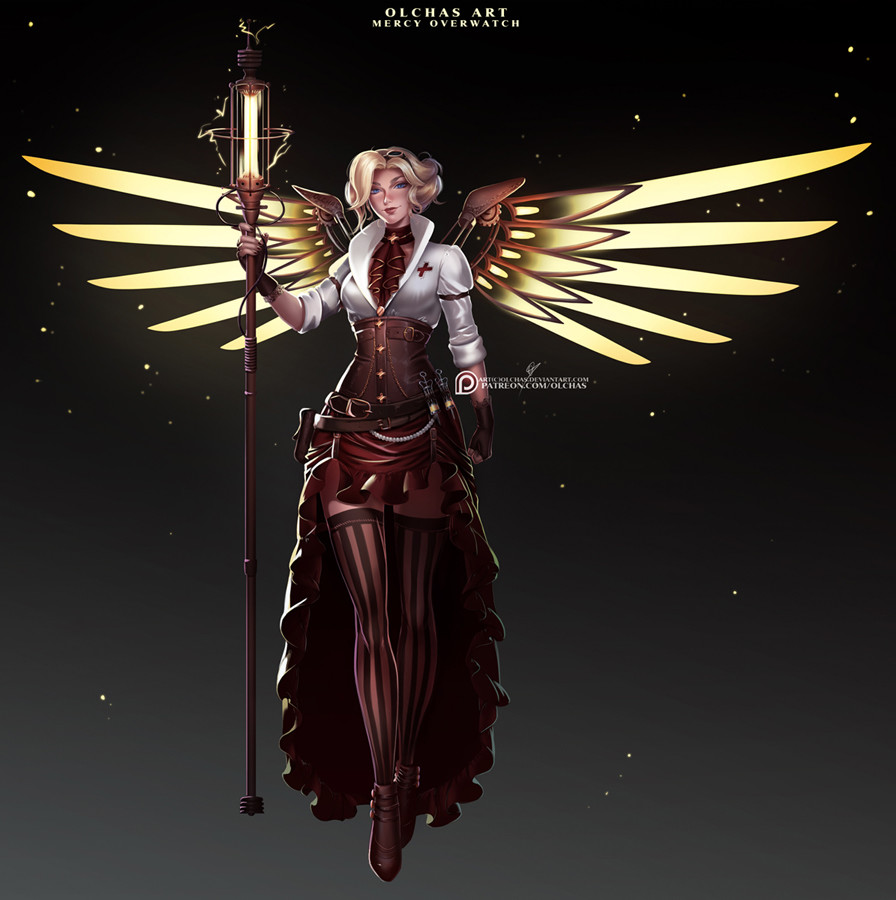The image is a detailed digital illustration featuring a central figure with a fantastical, fairy-like appearance. This woman, positioned in the center of the image, is adorned with golden, wing-like extensions on her back and has short blonde hair. She is holding a maroon staff that culminates in a glowing, yellow torch. Her outfit consists of a maroon gown with a white top, featuring a large lapel and a plus symbol on the chest area. Additional details include red pants and black tights, contributing to her intricate and striking attire. The background of the illustration is black, adorned with scattered white and yellow stars, creating a celestial ambiance. There is white text that reads "Olka's art" prominently displayed at the top of the poster. This digital art piece carries a strong resemblance to video game or cartoon character design, complete with a blend of mysticism and detailed craftsmanship.